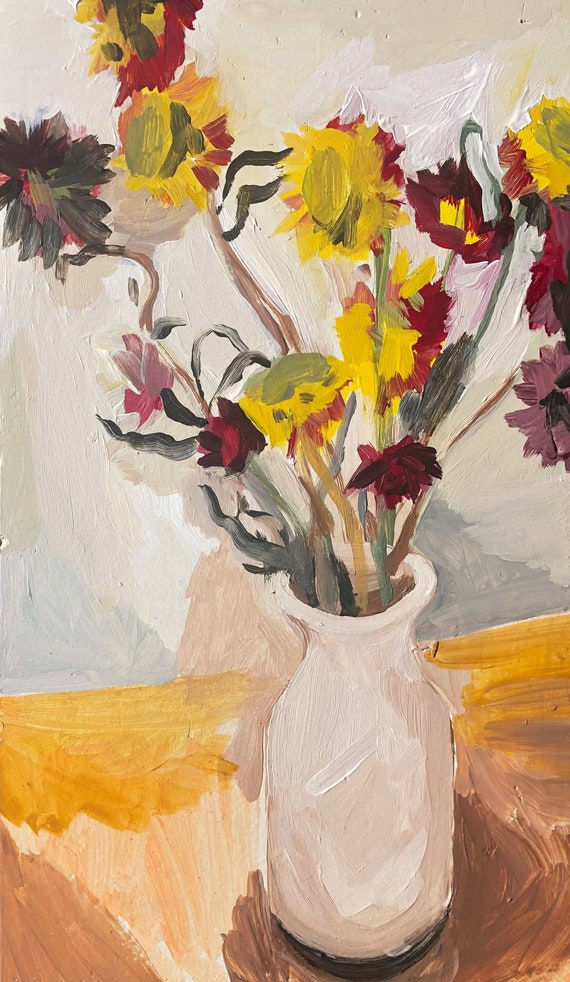The painting, likely a watercolor, presents a vivid and tall composition of a simple table with a vase of flowers. The table, understated and rendered in shades of brown and yellow, serves as a foundational element but lacks intricate detail. Central to the scene is a white vase, shaped reminiscently like a milk bottle, tall and narrowing at the top before flaring out to cradle an array of blooms. The flowers, a lively assortment of large yellow and red blossoms interspersed with occasional magenta ones, extend energetically in various directions. Some yellow flowers resemble smaller sunflowers with green centers, whereas the darker red flowers feature yellow centers, with a purple flower adding contrast to the right. These blooms, while identifiable, lack fine detailing, emphasizing broad brushstrokes over precision. The background wall is understated in a light shade of grey, with hints of faint blues and pinks blending softly into each other, capturing subtle shadows cast by the vibrant bouquet.